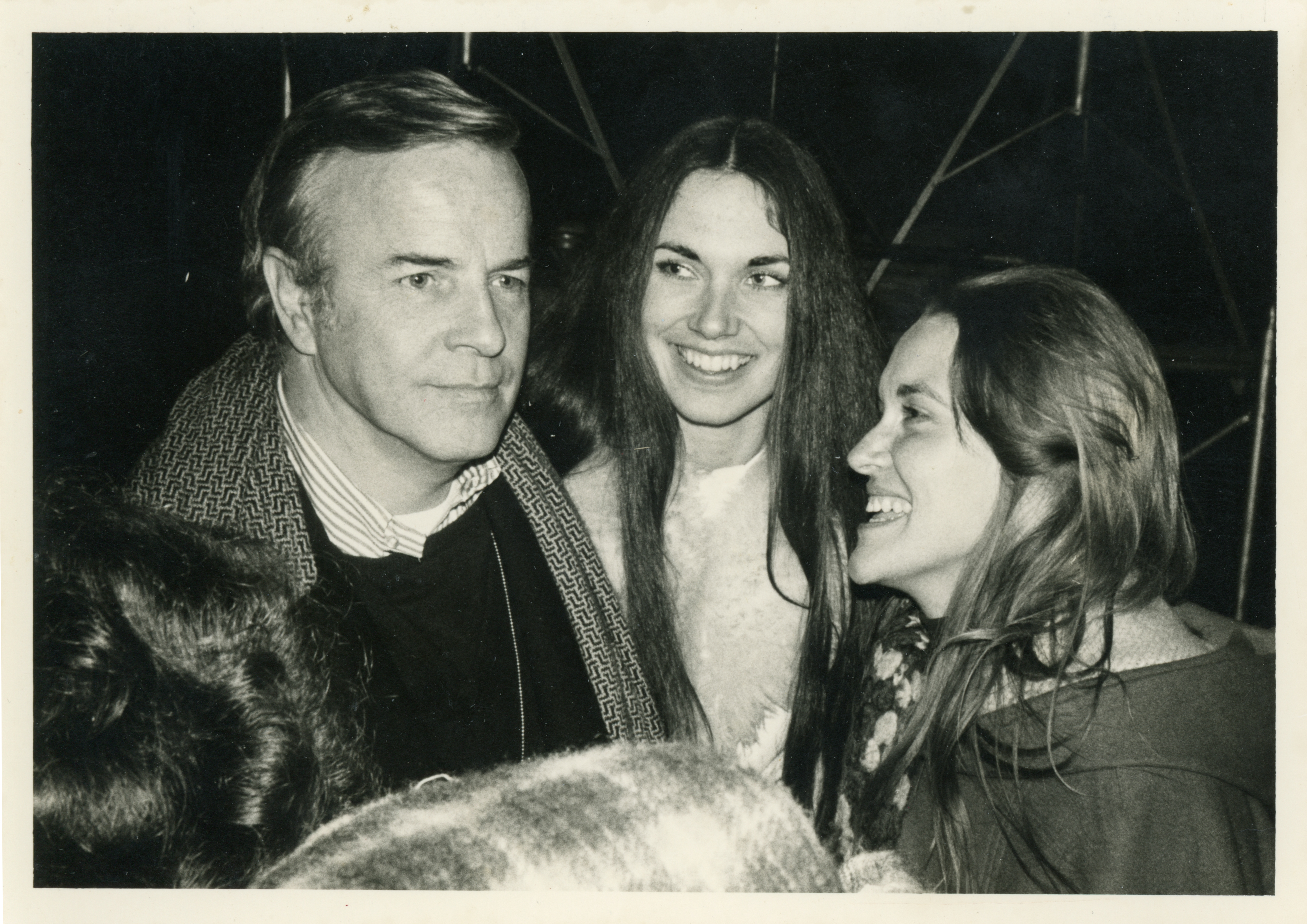This black-and-white photograph, possibly from the late 1960s or 70s, captures an outdoor scene with a middle-aged man and two women, all dressed warmly in jackets, suggesting a chilly day. The man, around his 40s, has a high forehead and a slight smile, and is dressed in a black striped shirt paired with a scarf. His face is turned, gazing towards the lower right corner of the image. To his right stands a young woman with long black hair reaching nearly to her waist. She is smiling gently, her head subtly turned towards the man as if they are engaged in conversation. Beside her is another woman, shorter in stature with light brown hair falling just past her chest. She is also smiling and looking at the man. Both women wear coats, and the second woman has a scarf. The dark, gray background is punctuated by blurry, shiny elements in the foreground, possibly someone's hair or a reflective object. Tree branches in the background further suggest an outdoor setting. In the lower left corner, a fourth individual’s head is partially visible, adding a mysterious element to the scene.